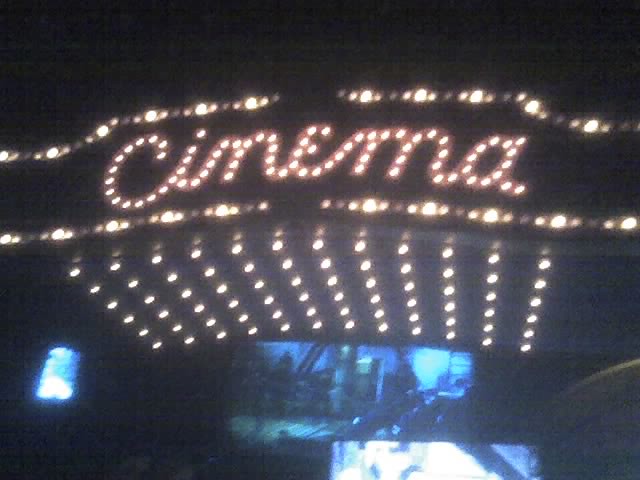The image features a dreamy, nighttime outdoor setting at a movie theater. The central focus is a large, illuminated sign with LED bulbs that spell out the word "cinema" in cursive. The bulbs form strings of lights at the top and bottom of the text, casting a warm yellow, light blue, and white glow against a predominantly black background. Below the sign, there are several TV monitors or screens, though they're slightly blurry, creating an almost surreal atmosphere. The overall effect is an inviting, cinematic ambiance, combining nostalgia and modernity through its luminous display.